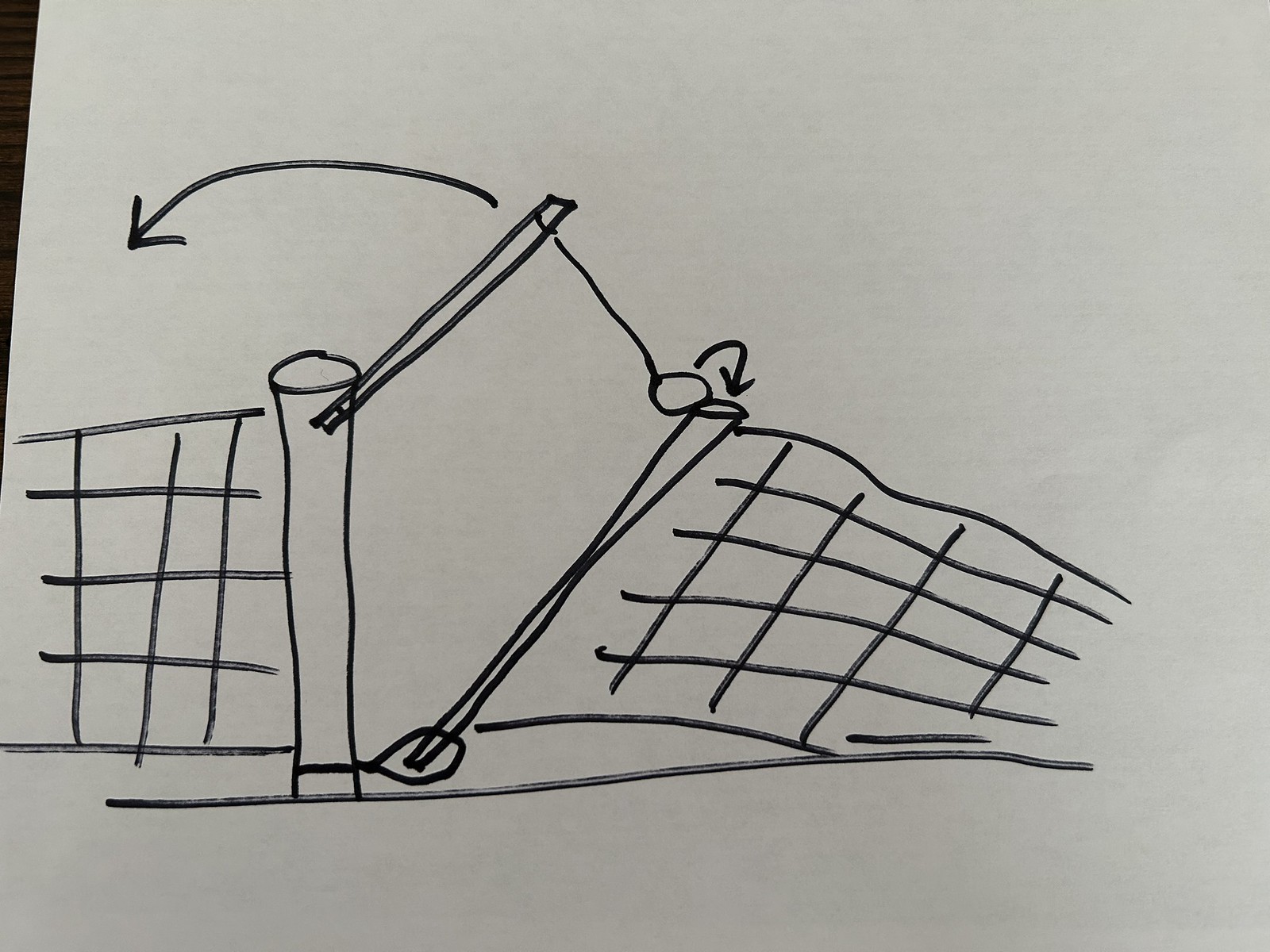This photograph captures a white piece of paper with a detailed black Sharpie drawing, illustrating the potential construction of an articulated fence. The line drawing features vertically and horizontally cross-hatched sections that appear connected to a central post. At the base of this post, there is a connection point leading to another section of the fence that is depicted as leaning over, resembling the structure of a volleyball net. Various arrows and annotations indicate the connections and pivot points, suggesting how these fence sections might be attached to the central post. The drawing conveys a design concept where the fence could be lowered or articulated for easy access, showcasing a practical and flexible mechanism.